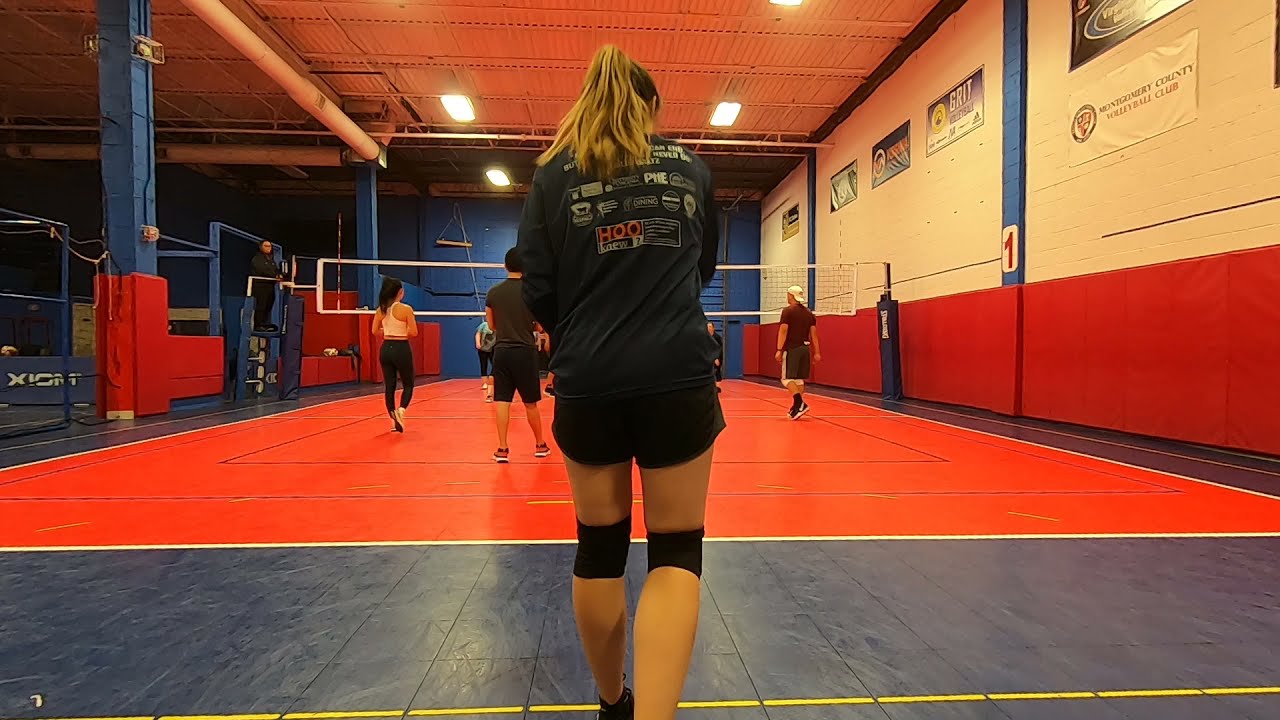This detailed image captures an indoor volleyball game taking place in a gym. The gym's walls have a cream-colored upper section with a red lower border, accentuated by blue horizontal lines, and adorned with various banners. A white sign with a red number "1" indicates this is court number one. The flooring of the gym is separated into a multicolored volleyball court, with a reddish-orange play area bordered by a blue outer region.

In the center foreground, a blond woman wearing a dark shirt, dark shorts, and knee braces stands with her back to the camera, poised to serve the ball, which is inferred to be in her hands. She stands on the blue section of the court, indicating her position in the game. Stretching across the image is the volleyball net, with indistinct players visible on either side, emphasizing the co-ed nature of the match. To the left, a person is elevated on a platform, likely officiating or overseeing the game. The platform and surrounding barriers are also color-coordinated in red and blue, with sturdy blue pillars providing support. The gym floor, possibly made of a rubber protective cover, highlights the anticipatory moment within this recreational volleyball environment.